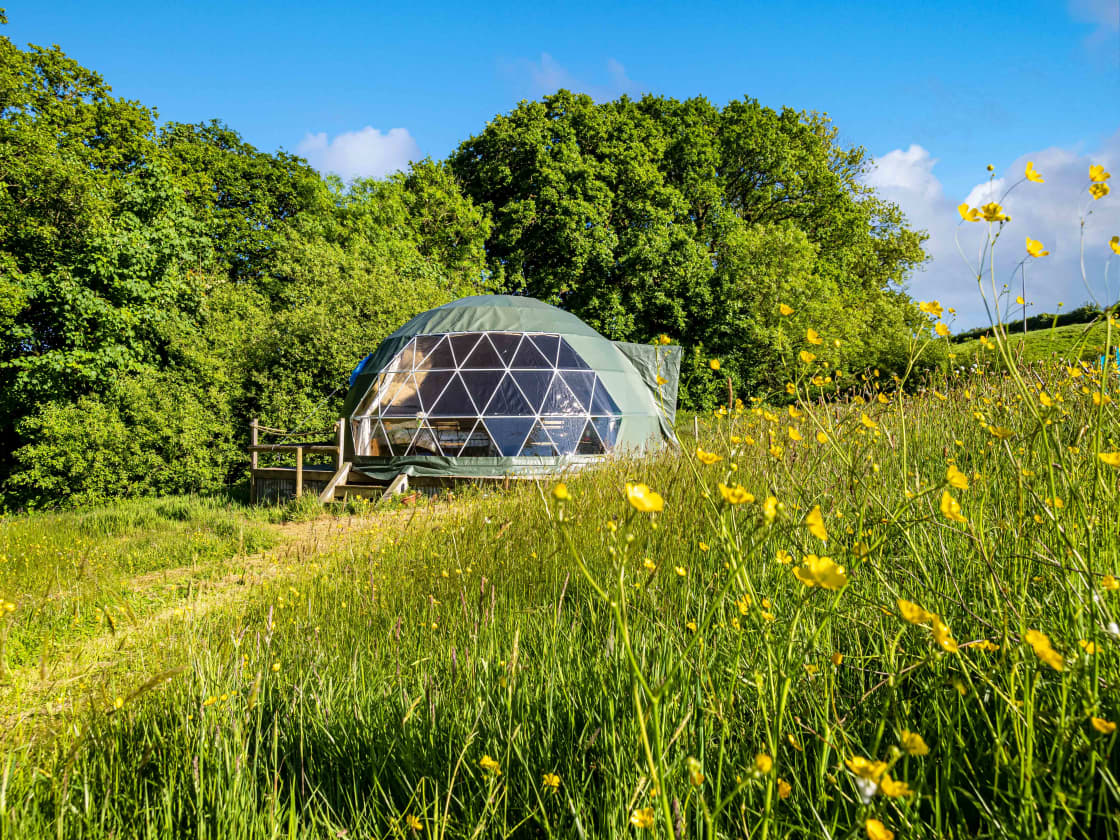The image features a high-tech, semi-circular polyhedral tent situated in an outdoor wilderness area, surrounded by nature. The tent, which appears green at the base with transparent triangular windows making up the front, is anchored with ropes and includes wooden steps leading up to a small porch. It is nestled amidst a variety of greenery: a grove of trees frames the scene to the left and right, offering protection against the elements. A worn pathway, originating from the lower left corner, winds through a grassy field dotted with numerous yellow flowers and leads up to the tent. The backdrop showcases a serene blue sky adorned with fluffy white clouds, suggesting it is taken during the daytime, possibly mid-evening. The sunlight illuminates the scene from the right, casting a gentle glow over the vibrant landscape.